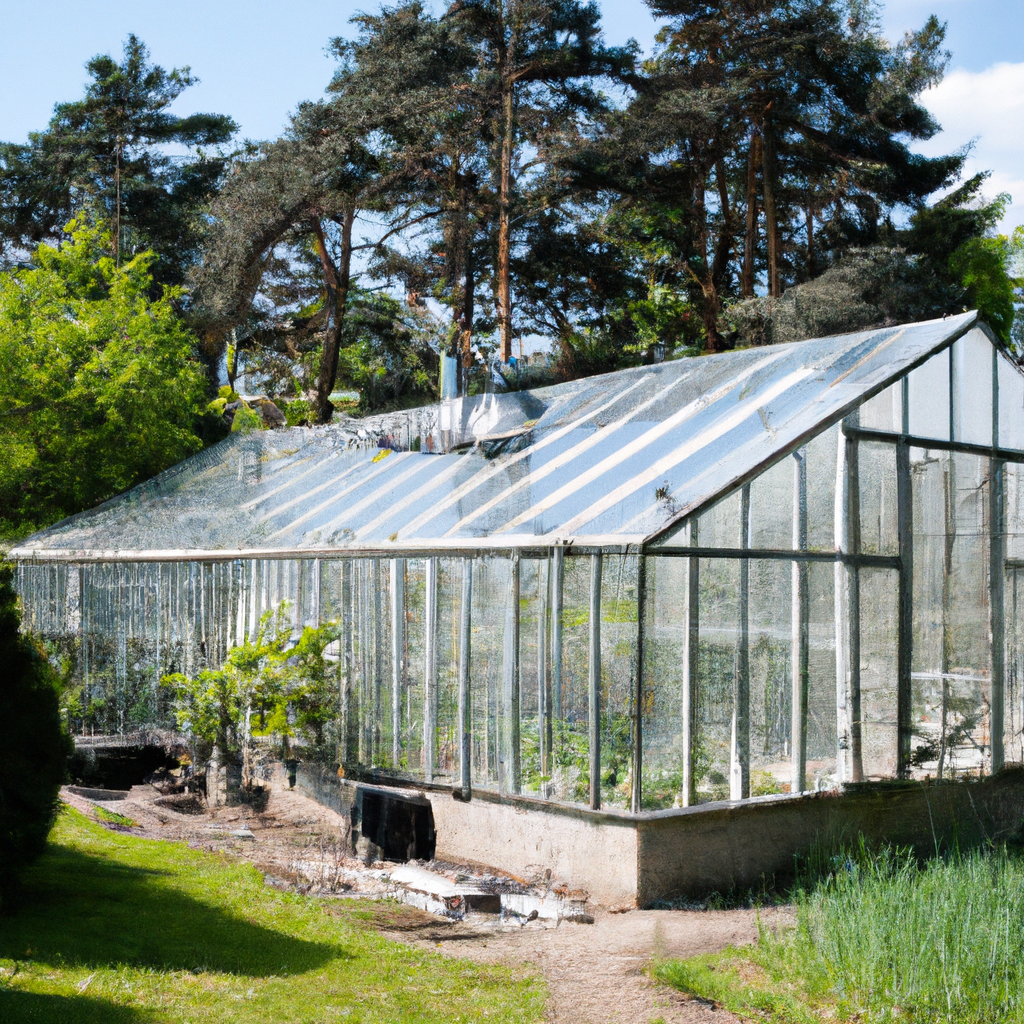The photograph depicts an outdoor scene during the daytime, showcasing a medium-sized, square-shaped greenhouse, approximately 5 to 6 inches in height and width in the image. This transparent greenhouse, possibly made of glass or plastic, features a triangular, sloping roof with metal rods for support, and visible plants inside through the clear windows. Notably, at the top center of the structure, there is a damaged area or a purposeful opening to allow sunlight in. 

The vantage point is from a corner, allowing a view of both the left and right sides of the greenhouse. On the left side, there is a neatly mowed patch of grass, while the right side has overgrown grass, suggesting a deliberate choice to let that area grow. Beside the greenhouse, a small pathway extends toward and then around it. Surrounding the structure, there are several trees with brown trunks and green leaves, and bushes that might include tomato plants. The background is filled with tall trees and a blue sky adorned with a few white clouds.